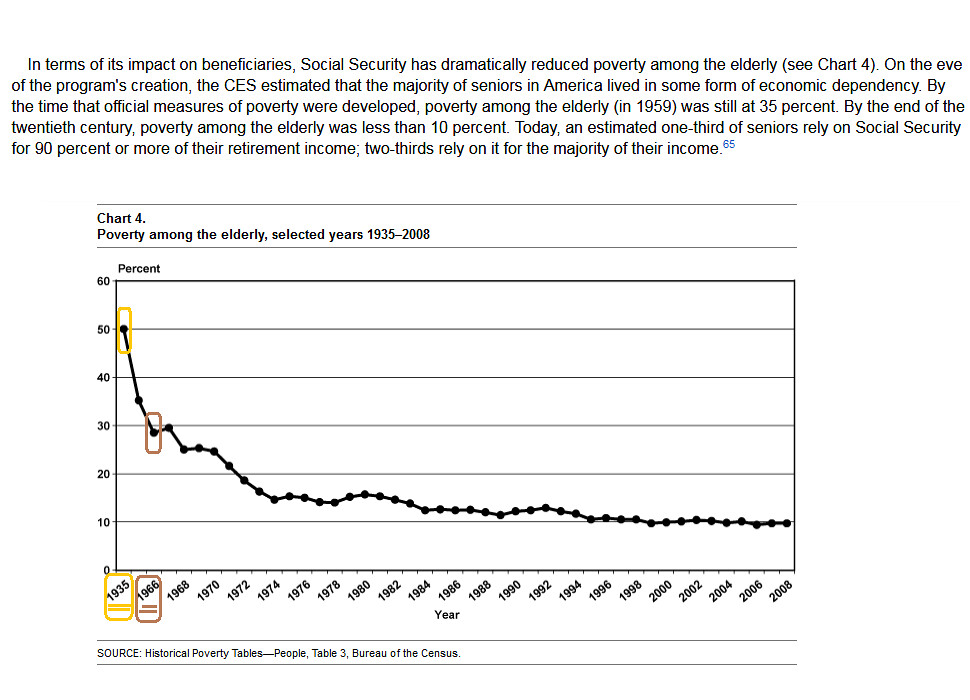The image depicts a line graph titled "Poverty Among the Elderly, Selected Years 1935 to 2008," with annotations emphasizing the significant impact of Social Security on reducing elderly poverty. The graph, labeled as Chart 4, features a vertical axis ranging from 0% to 60% and a horizontal axis spanning from 1935 to 2006. In 1935, 50% of seniors lived in poverty, but this figure trended downward dramatically over the decades. By 1959, poverty was at 35%, and by the 1990s, it had stabilized around 10%, reaching its lowest point by 2008. Accompanying text explains that before Social Security's inception, the majority of American seniors were economically dependent. By the end of the 20th century, the poverty rate among the elderly had dropped to less than 10%. Today, Social Security is a crucial source of income, with one-third of seniors relying on it for 90% or more of their retirement income, and two-thirds for the majority of their income.